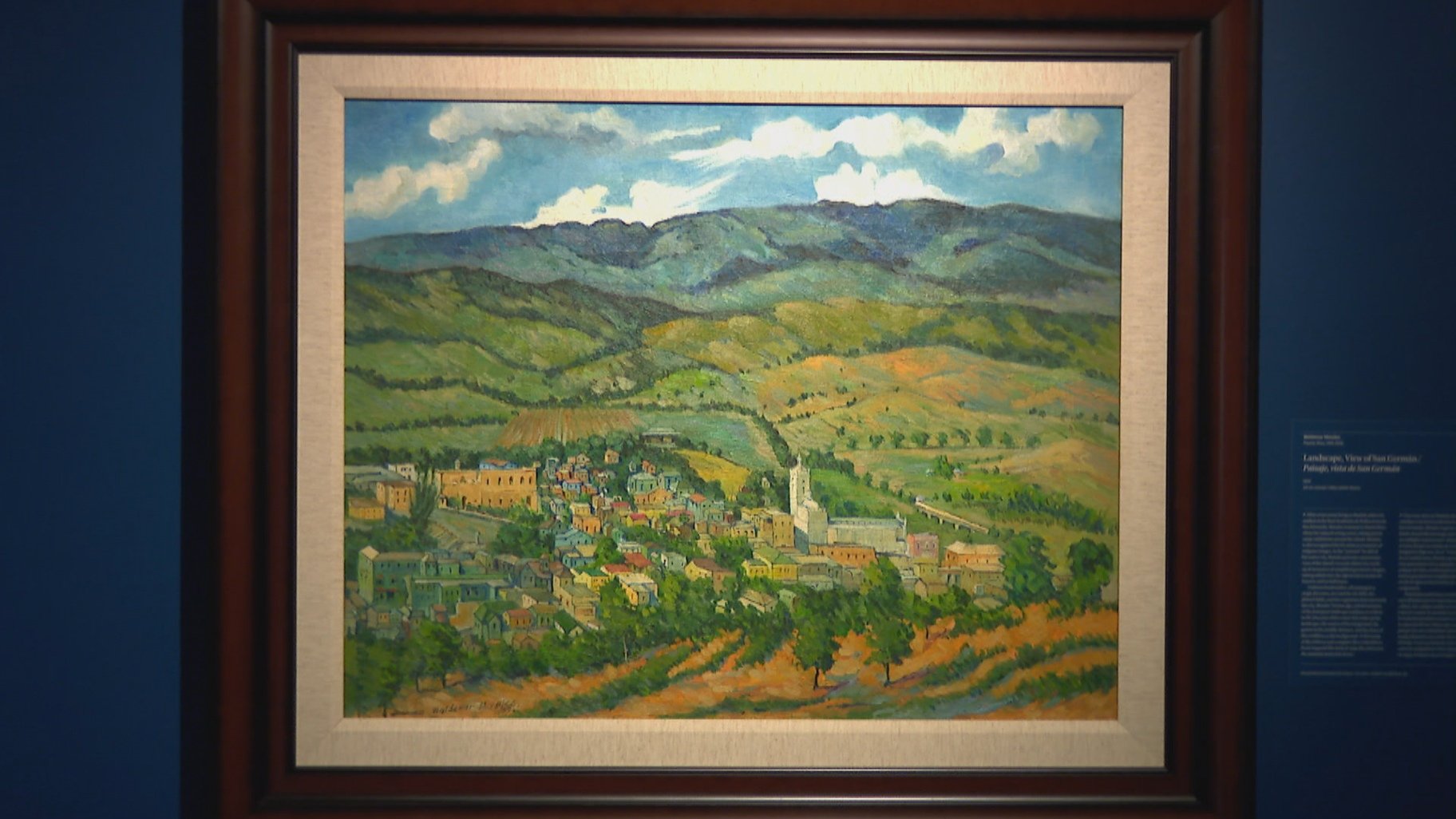This image captures a detailed painting prominently displayed in a museum or art gallery. The painting, surrounded by a dark brown wooden frame accented with a lighter gray matting, depicts an intricate Italian countryside scene. The foreground features a variety of tall, bushy trees growing from earthy, orange-brown soil. Nestled among the greenery are buildings of various colors—some with red, blue, white, and green roofs—that form a quaint village. Prominent among these structures are a picturesque church and a castle-like building surrounded by what appears to be ancient city walls. 

Further into the picture, cultivated farmland stretches behind the town in neat rows, adding to the pastoral charm. The hills beyond the village rise gently, adorned with more trees and golden grasses before culminating in green and gray mountains. The scene is set against a backdrop of an expansive blue sky dotted with big, fluffy white clouds. 

To the right of the painting, on the blue wall of the gallery, is a piece of paper or a printed document, presumably detailing information about the painting and the artist, though the text is too small to discern in the image. The entire composition immerses the viewer in a serene and harmonious blend of natural beauty and quaint village life, typical of an idyllic countryside landscape.